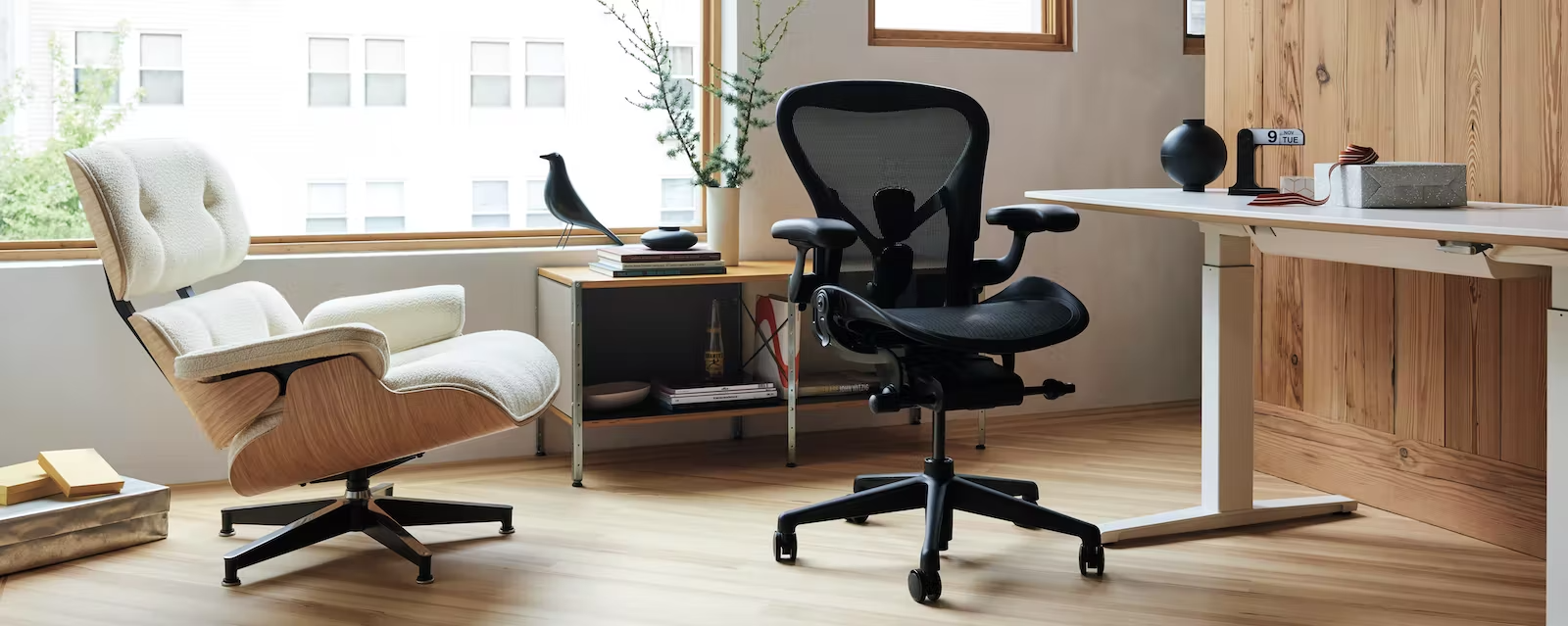This photograph captures a meticulously decorated office space, potentially a home office, bathed in natural light streaming through a window overlooking another building with glimpses of green trees outside. Centered under the window is a compact book table adorned with a few stacked books, a black statue of a bird gazing outside, and a white vase filled with green foliage. The room features a blend of neutral tones with subtle hints of blue and green.

The seating arrangement includes two distinct chairs: an off-white reclining chair with a delicate beige underside and soft, inviting texture positioned to the left, and a functional black office chair with adjustable height on the right. Both chairs are equipped with wheels for easy mobility.

To the far right of the image is a sleek, modern white desk placed against a vertical plank wall with wide, light-colored hardwood. The desk surface hosts a few indistinguishable items, including a black vase, adding to the minimalist aesthetic. The background reveals a white wall with light brown trimmed windows, blending harmoniously with the beige paneling of the vertical plank wall, creating a cohesive and warm environment.